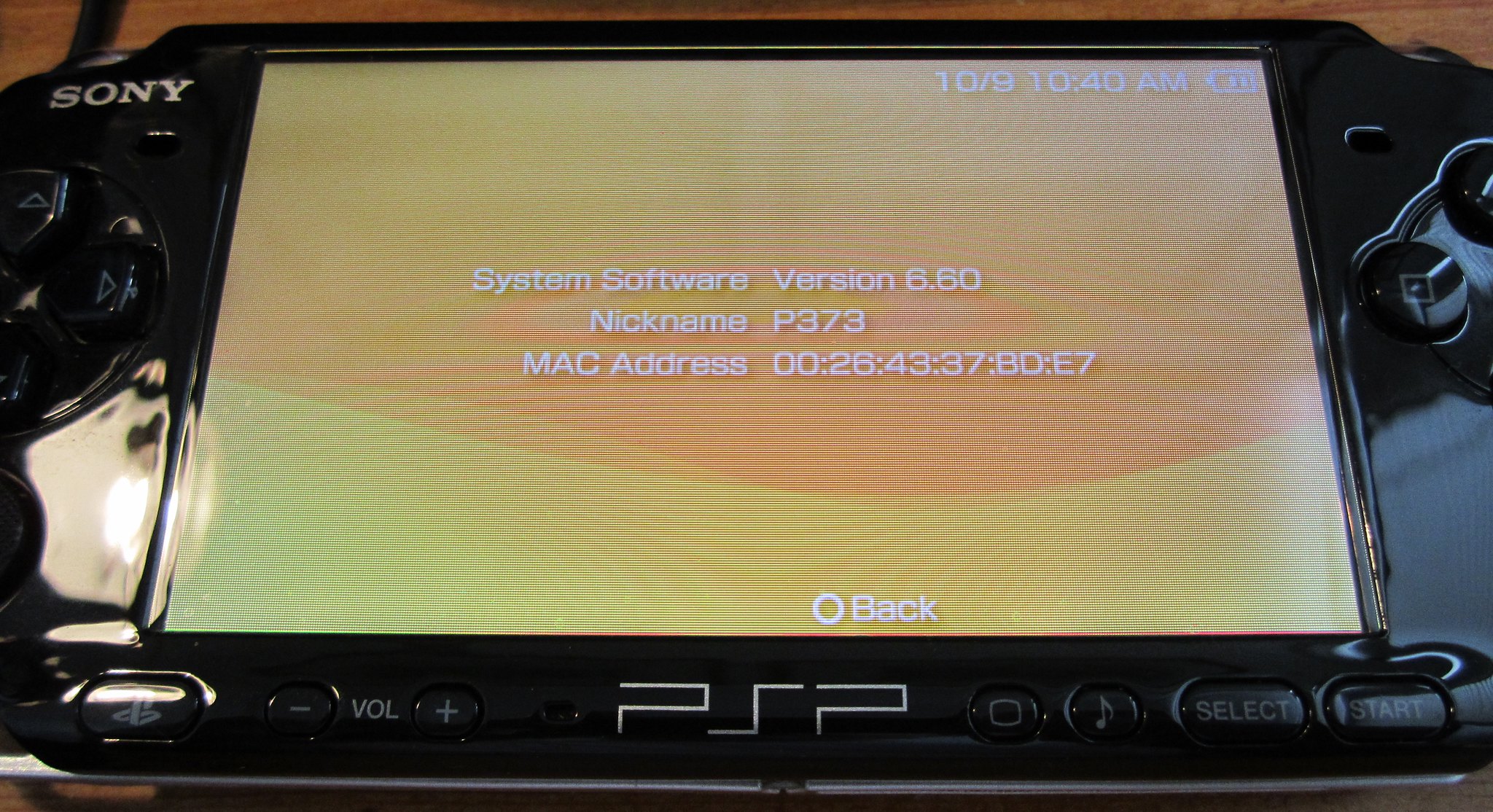This image showcases a black PSP (PlayStation Portable) handheld gaming console prominently displayed on a surface, occupying the entirety of the photo. The PSP features a substantial screen for its size, displaying a yellow-themed interface. Text on the screen indicates details such as the date and time (10-09, 10:40 AM), System Software version 6.60, nickname P373, and its MAC address 0026433780E7. The console is equipped with various controls, including a D-pad (up, down, left, right), volume buttons, Bluetooth link, music mute, and action buttons (square, triangle, circle, and X) as well as 'Select' and 'Start' buttons positioned beneath the screen. The setting appears to be indoors, with overhead lighting highlighting the device's sleek black exterior and its multi-colored (orange, yellow, black, white, and gray) elements. The device is depicted lying flat on a tabletop, emphasizing its portable and compact design.